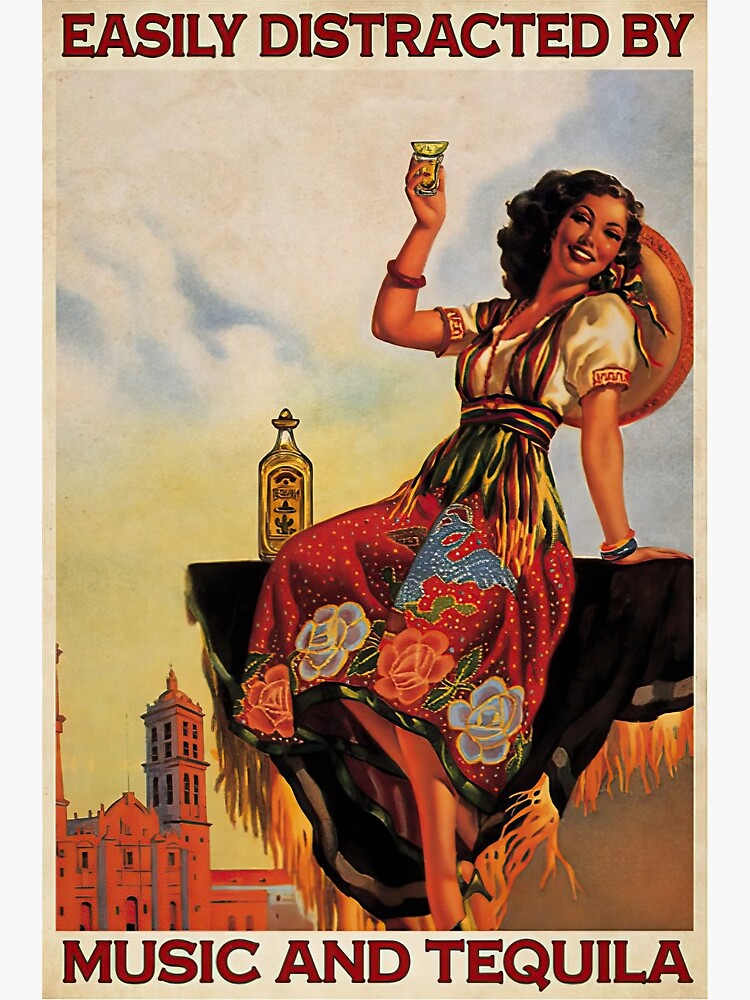The poster, printed on tan paper, features an old-time advertisement style with a Mexican theme. At the top of the poster, it reads in capital letters, "EASILY DISTRACTED BY," while the bottom line says, "MUSIC AND TEQUILA." The central image showcases a woman dressed in festive Hispanic attire, which includes a white blouse with puffy sleeves, a waistband striped in red, green, and yellow, and a wide red skirt adorned with circular patterns of orange and blue flowers. A sombrero is tied to her back. She is sitting on the corner of a building or ledge, with a blanket draped over the edge and a bottle of tequila beside her. With her head tilted back in a smile, she raises a shot glass with a lime in a toasting gesture. The sky behind her is partially blue with scattered clouds.